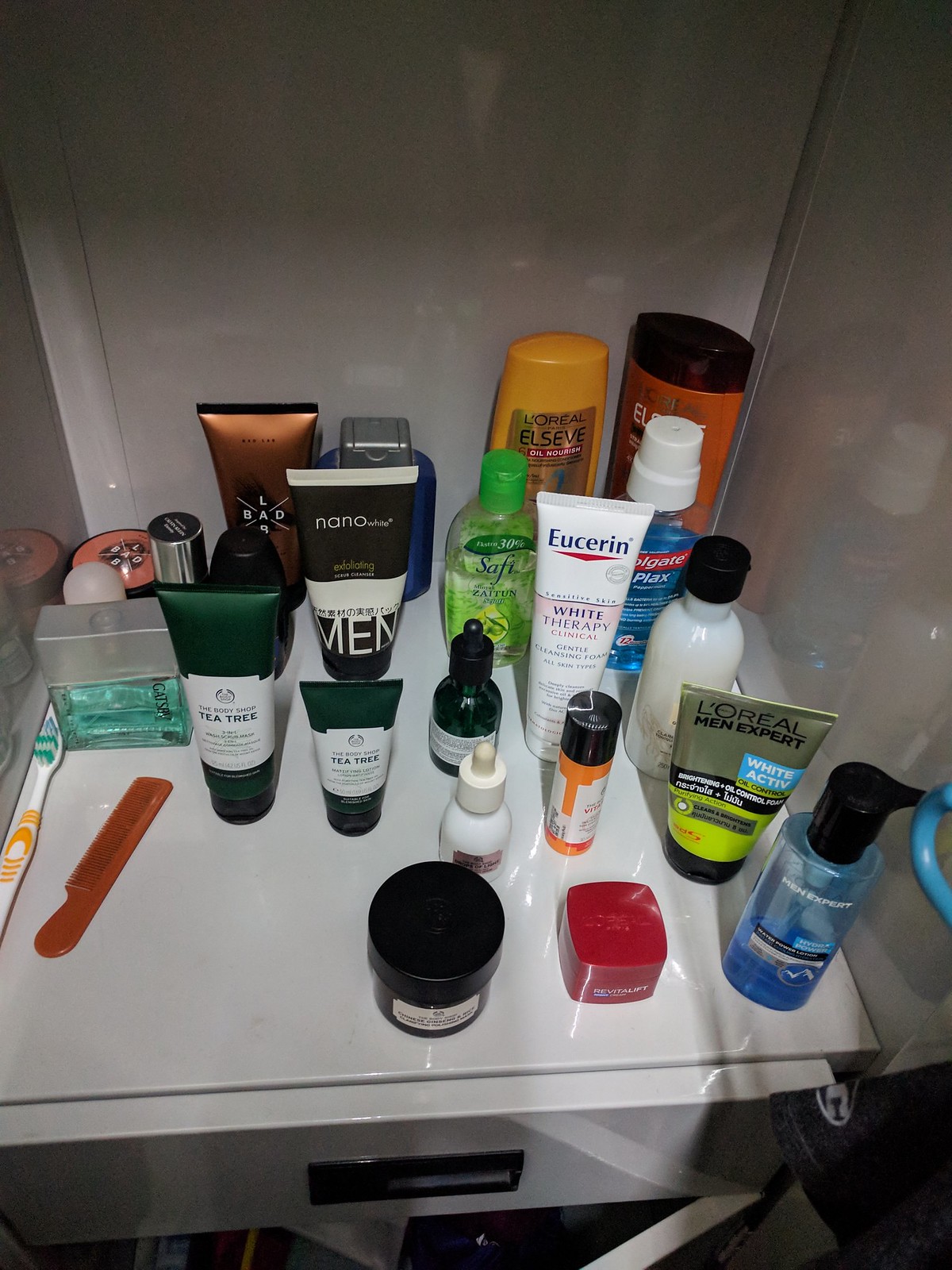This image showcases a makeshift shelf inside a bathroom closet, filled with a neatly arranged assortment of masculine toiletries. The dimly lit scene relies on light from an adjacent space, creating a subtle glow on the items. The "shelf" is actually the top of a white metal drawer unit with a black handle, adding a touch of functional simplicity.

On the left side of the drawer, we find a white toothbrush and a brown comb, essential items for daily grooming. Next to them sits a bottle of men's cologne, exuding an air of sophistication. Directly behind the cologne, partially obscured, are a jar and a compact item that could be a trial-sized deodorant.

Moving rightward, two tubes labeled "Tea Tree" suggest the presence of hair or skincare products. Behind these, yet another item labeled for men might be a shaving product, given the blue glass bottle behind it likely containing aftershave. 

Centered on the makeshift shelf are several tubes and a small black jar, their contents a mystery. Nearing the right side, a recognizable bottle of Eucerin lotion stands, adjacent to what appears to be hand sanitizer or a gel product in a pump bottle.

At the far right, nestled in the corner, is a L'Oreal shampoo conditioner, alongside a Colgate Plax mouthwash. Completing the collection, an item from the L'Oreal Men Expert range and another bottle with a black pump suggest more hair or skincare solutions.

This organized array of toiletries, spanning from dental care to grooming products, offers a comprehensive look at a man's daily hygiene essentials, all thoughtfully stored atop a drawer repurposed as a convenient shelf.